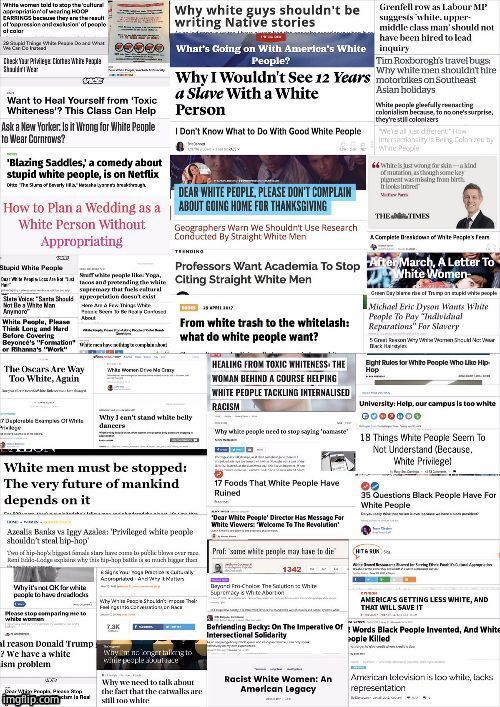The image depicts what initially appears to be a news website, but upon closer inspection, it becomes evident that it is a collage of various headlines, seemingly clipped together from online articles. The headlines, primarily focused on themes of race and particularly critical of white people, are arranged in three main columns, with a fourth narrower column at the bottom. Most headlines are presented without accompanying photos. Some of the discernible headlines include:

- "How to plan a wedding as a white person without appropriating"
- "White men must be stopped, the very future of mankind depends on it"
- "We need to talk about the fact that catwalks are still too white"
- "Racist white women and American legacy"
- "American television is too white, lacks representation"
- "From white trash to white lash, what do white people want?"
- "What's going on with America's white people?"
- "Politicians want academics to stop citing straight white men"
- "America's getting less white and that will save it"

The collection of headlines appears to reflect a critical and somewhat contentious perspective on whiteness and race relations in contemporary society. The mood conveyed by the collage is provocative, sparking thoughts on issues of racial dynamics and societal changes.